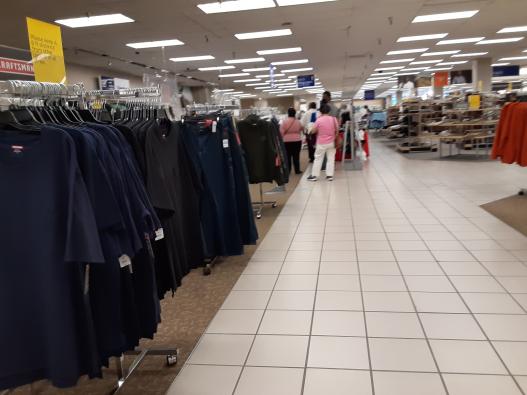The image is a poorly taken, low-quality photograph of the inside of a department store, viewed from the central walkway. The floor is covered with off-white or light beige tile, and the ceiling is lined with rectangular fluorescent lights, extending into the distance. On the left side, there is a prominent sign that reads "Craftsmen," indicating a possible toy department. Below this sign, we see racks of men's clothing, including blue and black shirts, pants, and what appears to be turtleneck pullover hoodies.

Further along the left side, there is a red and white sign, blurred and unreadable, above more rows of dark-colored clothing that include t-shirts and possibly jeans, all hanging on metal rods. Two women are waiting in line. The woman in the back is wearing khakis, dark sneakers, and a pink short-sleeve shirt, holding a handbag. She has dark hair that may be pulled back. In front of her, slightly to the left, is another woman also wearing a pink shirt with a handbag slung over her right shoulder, dark pants, and dark shoes. Another person in the forefront wears a white long-sleeve top, possibly a sweater or coat. On the right side of the image, there is a cropped rack displaying red long-sleeve shirts. Beyond this, the walkway seems to lead into another section that appears to sell shoes or other non-clothing items.